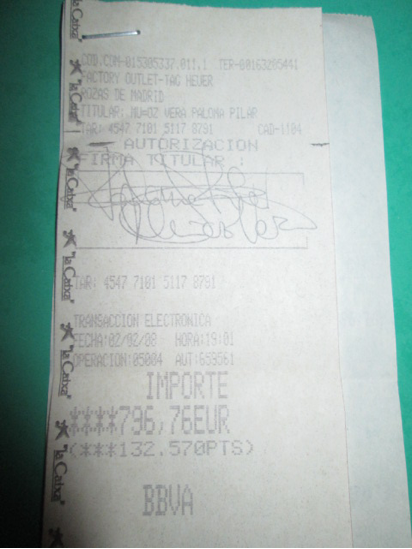The image showcases a close-up view of a receipt written in Spanish, featuring very dim ink that makes it difficult to decipher. The visible text includes phrases like "factory outlet," "IMPARTE," and "BBVA," along with various numbers, including "132.570 PTS." There are signatures present, possibly two on separate lines. The receipt is stapled to another, slightly wider piece of paper or receipt, whose text is not visible. Both are attached to a seafoam green or teal-colored background, which transitions from lighter to darker shades. The exact nature of the attachment is unclear, as it's uncertain whether the staple secures the papers directly to the teal background or just to each other.